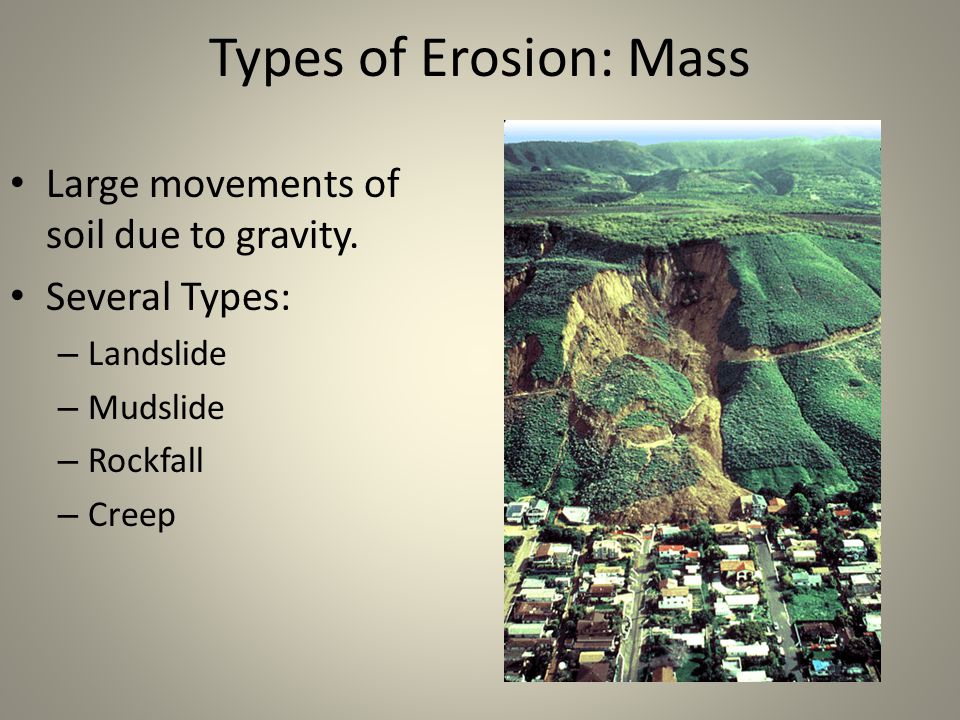This image depicts a PowerPoint slide with the title "Types of Erosion: Mass" prominently displayed at the top against a grey background. On the left side of the slide, black text details the various types of mass erosion, including "large movements of soil due to gravity" and enumerates specific types: landslide, mudslide, rockfall, and creep. On the right side of the slide, an image illustrates a hilly or mountainous environment where erosion is visibly taking place. In the image, light brown soil is exposed as grass and vegetation have been displaced by the downward movement of earth, revealing bare patches on the hillside. A residential neighborhood is depicted at the bottom of the slope in a valley, with several brown and white houses some of which appear to be partially submerged by the fallen soil. The landscape also features a blue sky, green areas of grass, and various other colors including black, tan, and red, further emphasizing the natural setting and the impact of erosion.